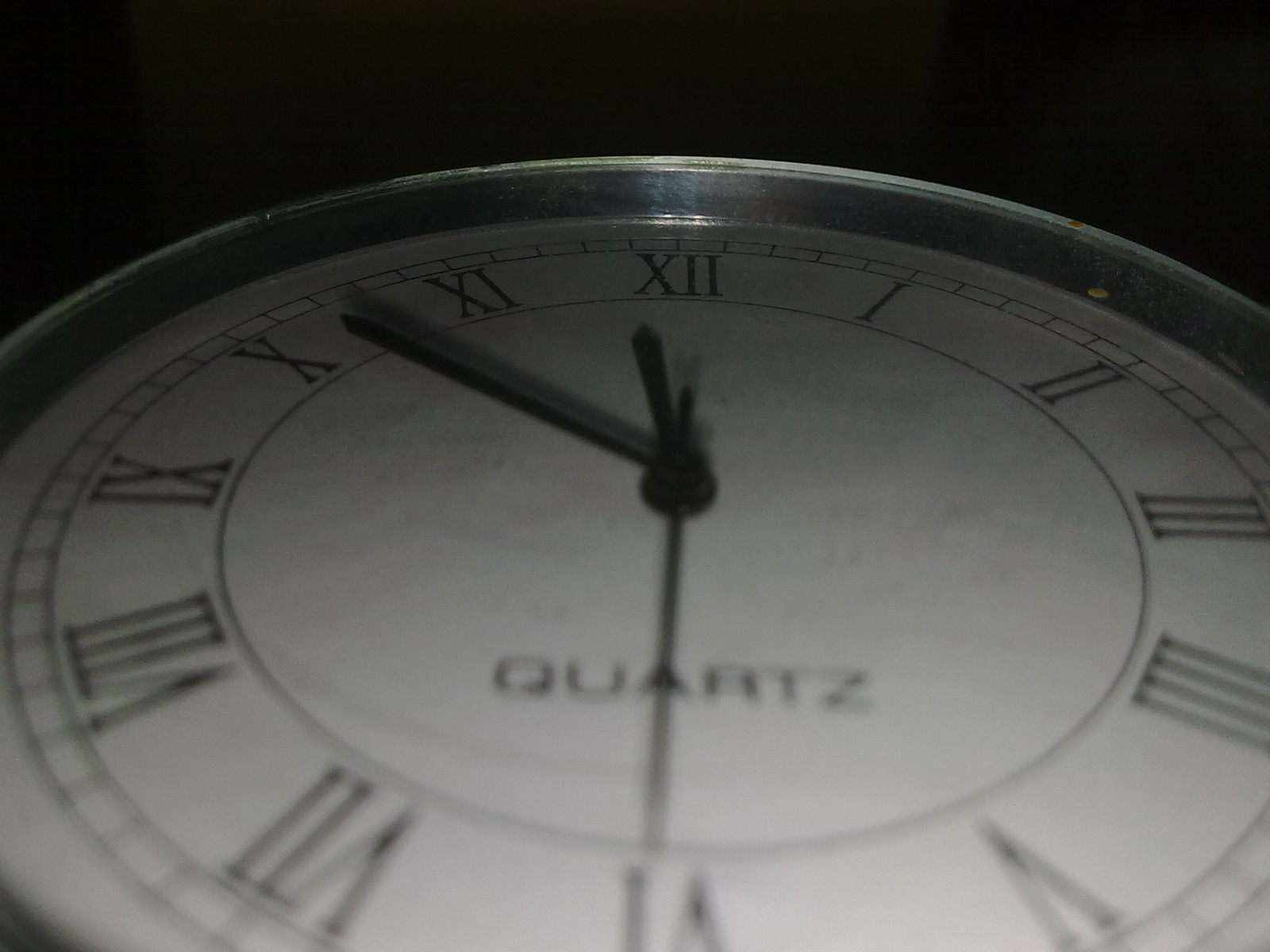The close-up image depicts the face of a white quartz clock, set against a starkly black background that suggests a dimly lit or nighttime environment, likely illuminated solely by the camera flash. The face of the clock, encased in a silver rim, prominently displays the hours in bold black Roman numerals from I to XII. The minute, hour, and second hands are also black, with the second hand steadily ticking towards a time of approximately 11:53. The term "quartz" is inscribed at the lower part of the clock face, indicating the clock's make. Minute intervals are marked by small lines encircling the clock edge. The positioning of the clock suggests that it is resting or leaning at a slight angle rather than being mounted on a wall or worn on a wrist.